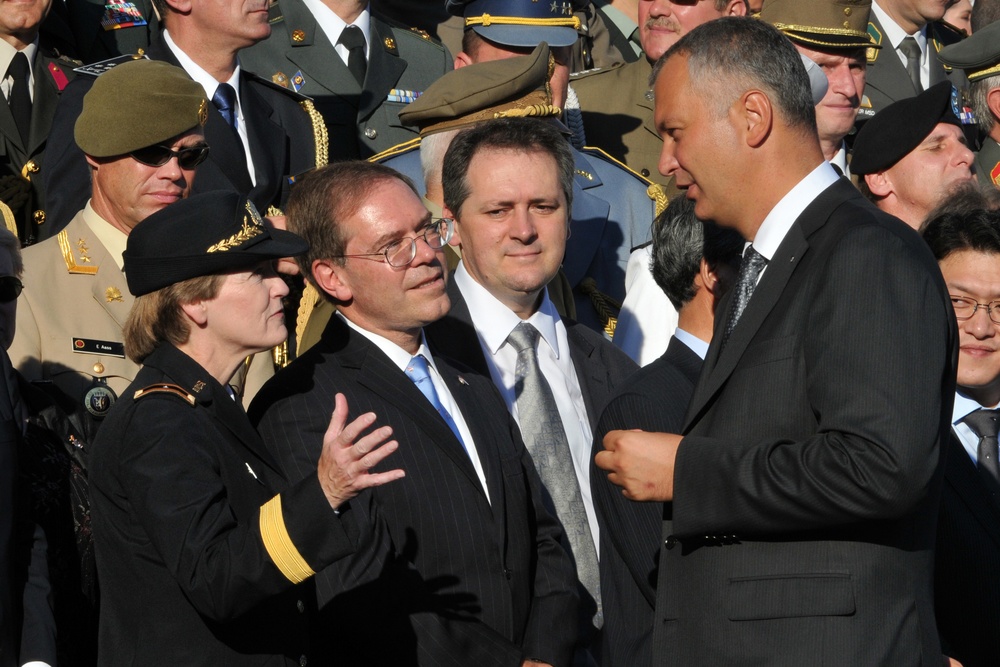The photograph captures a group of individuals, both military personnel and civilians, gathered outdoors on a sunny day. In the foreground, a semicircle of four central figures are engaged in conversation. On the far right stands a tall man in a black suit, viewed in profile, with short hair that is gray at the temples. To his left, another man, shorter in stature, wears a black pinstripe suit and a blue tie, and has glasses. Between them is a third man in a dark suit with a light shirt and gray tie, seemingly observing the interaction. On the far left is a woman in a military uniform, distinguishable by her black hat with gold leaves around the brim and a yellow band on the cuff of her dark jacket.

Behind this central group, several rows of military personnel fill the background, appearing to stand on bleachers or elevated platforms. These individuals are dressed in various military uniforms, indicating different branches and ranks. Some wear berets, others have hats with bills, and their uniforms range from darker greens to lighter shades, adorned with badges and name tags. The entire assembly is bathed in sunlight, as evidenced by the squinting faces and some people wearing sunglasses, all looking in a similar direction.